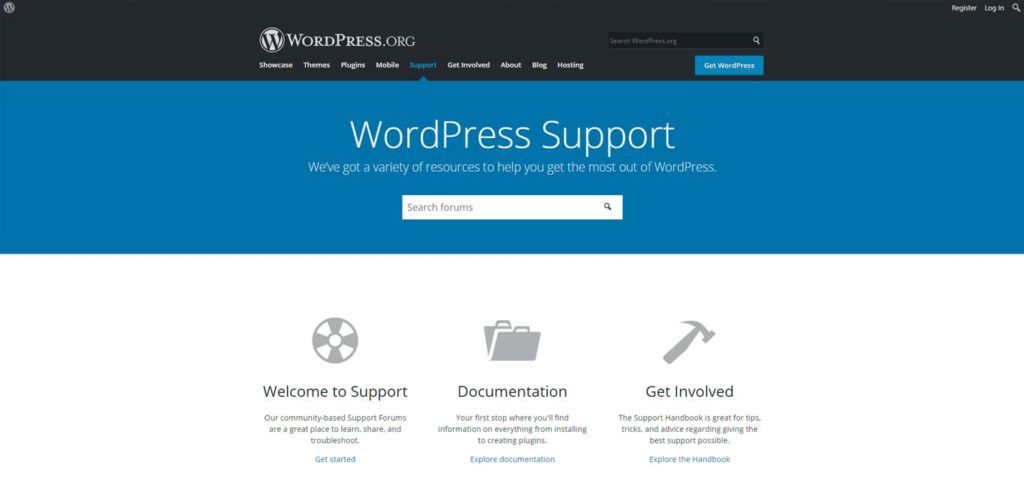The webpage displayed is from wordpress.org, featuring a sleek and intuitive design. At the very top, a thick black banner stretches across the width of the page. Positioned in the upper left corner of this banner is a white-gray circle with a black "W" at its center, signifying the WordPress logo. On the far right of the banner, in small white text, the options "Register" and "Login" are available, followed by a magnifying glass icon.

Just below this banner, prominent in the upper center of the page, the text "wordpress.org" is displayed alongside the WordPress logo. Adjacent to this on the right is a black search box. Directly beneath this header area is a horizontal navigation menu offering various options: Showcase, Themes, Plugins, Mobile, Support, Get Involved, About, Blog, and Hosting. The "Support" section is currently selected, indicated by a bright blue highlight.

The primary content area starts with a bright blue background. Centered in this section is bold white text stating "WordPress Support," accompanied by a subheading in smaller white text: "We've got a variety of resources to help you get the most out of WordPress." Below this, there's a white search box for browsing the forums, emphasizing the support aspect.

Following this introduction, the main content area on a white background showcases three icons arranged horizontally:

1. **Grey Gear Icon:**
   - **Label:** Welcome to Support
   - **Description:** Our community-based support forums are a great place to learn, share, and troubleshoot.
   - **Call to Action:** Bright blue text: Get Started

2. **Blue File Folder Icon:**
   - **Label:** Documentation

3. **Yellow Hammer Icon:**
   - **Label:** Get Involved